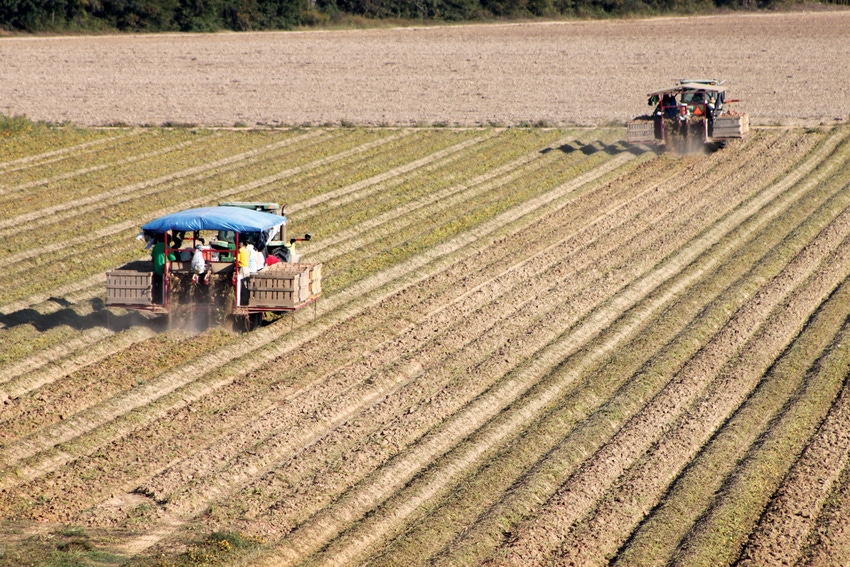The drone-captured color photograph, oriented in landscape, vividly depicts a field actively being harvested. The field, marked by furrowed rows running diagonally from the bottom left to the top right, showcases two tractors working in tandem, with one slightly ahead of the other. Each tractor pulls a trailer equipped with machinery, likely for digging up mounds of what appears to be potatoes, given the nature of the overturned soil and the rectangular mounds. Workers shaded under canopies—one blue, one beige—sort and place the harvested items into beige crates mounted on both sides of the trailers. The image, anchored by representational and realistic styles, shows the larger landscape with a dirt path set horizontally across the top and a backdrop of a plowed field and a green tree line. The field itself has a hint of green, possibly indicating young plants emerging amidst the rows.